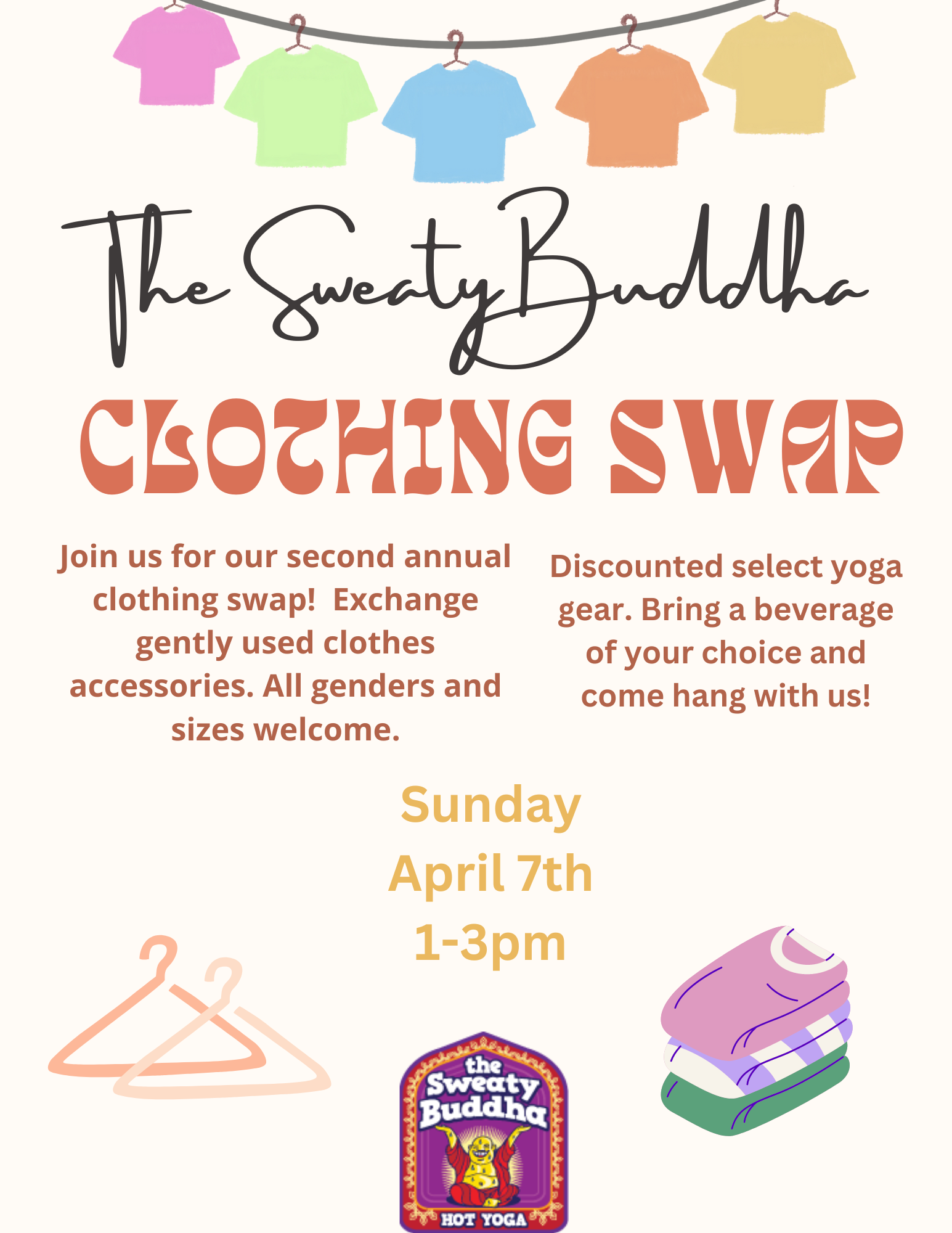This image features a detailed advertisement poster for an event organized by The Sweaty Buddha Hot Yoga studio. The poster’s background is a cream color and colorful elements adorn it. At the top, five short-sleeved shirts hanging on a clothesline are prominently displayed: from left to right, they are pink, light green, light blue, light orange, and light yellow.

In the center, the event title "The Sweaty Buddha" is written in black cursive text, and "Clothing Swap" is displayed in a reddish-orange text. Below it, the descriptive text in brownish-red reads, "Join us for our second annual clothing swap. Exchange gently used clothes and accessories. All genders and sizes welcome." On the right side, this same text color announces, "Discounted select yoga gear. Bring a beverage of your choice and come hang out with us."

A cartoon depiction of a yellow Buddha in a red robe, holding his hands up, is located in the middle of the poster, adding a whimsical touch to the advertisement. At the bottom left corner are two hangers, and the bottom right corner features folded clothes. Additional shirts are also showcased around these elements. The event details, "Sunday, April 7th, 1 to 3 p.m." are highlighted in yellow text. At the very bottom, the poster reiterates "The Sweaty Buddha Hot Yoga."